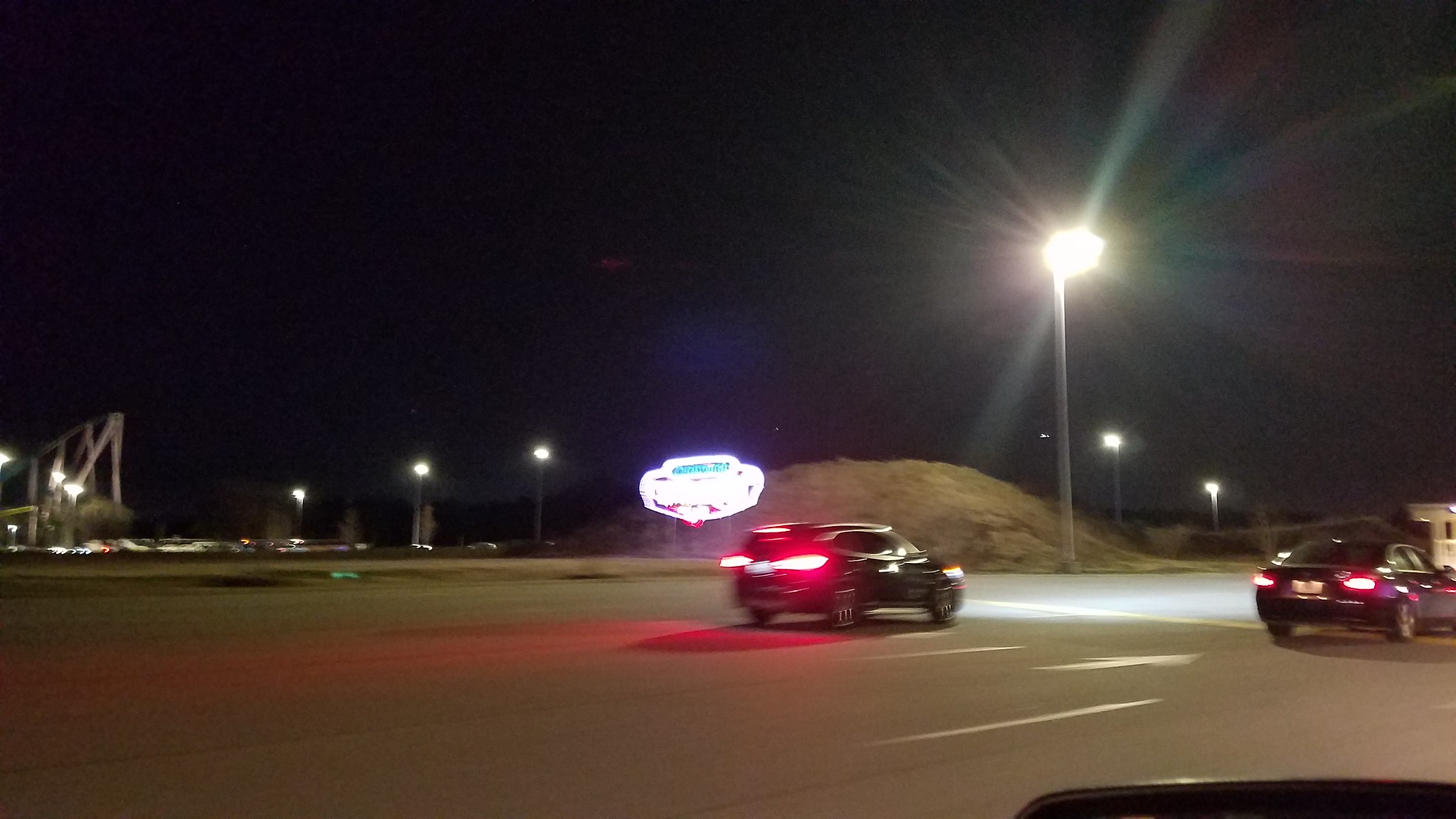The image captures a nighttime scene on a wide-open stretch of highway. Several cars, including a car and an SUV, are driving in the same direction on a multi-lane concrete road. Directly above the highway, a large streetlight beams down almost like a sun, illuminating the road with a bright, white light. The rear lights of the vehicles ahead are distinctly red. In the distance, additional smaller streetlights cast a faint glow.

To the left of the visible cars, a bright neon sign with an oval-shaped logo stands out, although the text is unclear. Adjacent to this, some trees and shrubbery can be seen, as well as what appears to be a hill or dirt mound with short brown grass. There is grass off to the left of the road, suggesting another lane possibly going in the opposite direction. A structure that resembles scaffolding or possibly part of a roller coaster is visible far in the distance, along with a crane-like artifact with long legs, situated above a car park. The night sky is a deep black-blue, encapsulating the scene in darkness.